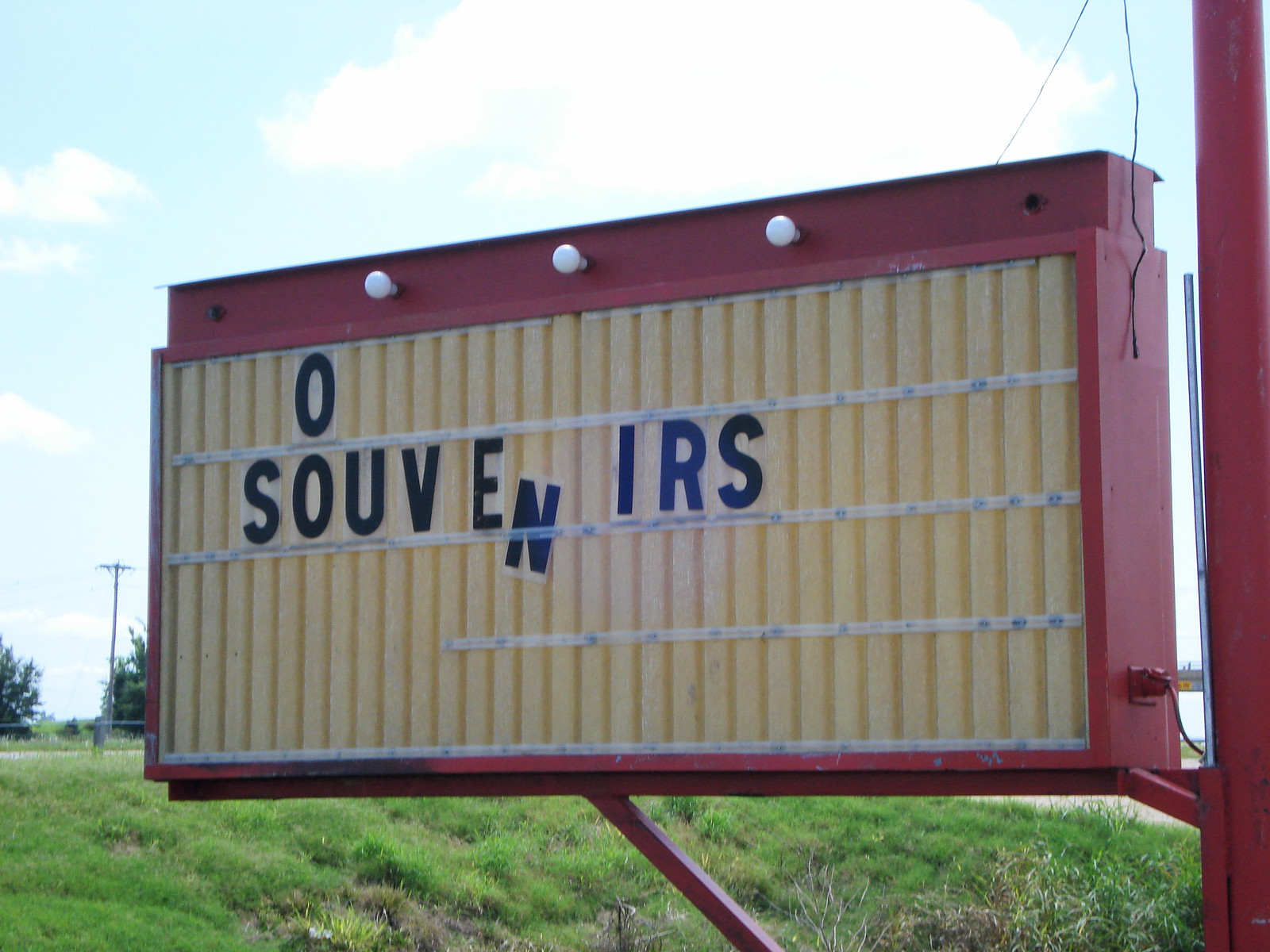The outdoor daytime color photograph showcases a close-up of a deteriorating sign, no longer in active use, with several letters missing or falling off. At the topmost line of the sign, only the letter "O" remains. On the second line, the word "Souvenirs" is partially intact, though the letter "N" has slipped behind a horizontal plastic holder, hanging at a slight diagonal due to dislodgment. The sign's red frame is adorned with three vintage Edison bulbs arranged in a row at the top, currently unlit, hinting that the sign was once illuminated to attract attention at night.

Below the sign, a grass verge with a steep gradient slopes upward towards the left, predominantly covered in green grass interspersed with patches of brown shrubbery. Above the sign, an overexposed, fluffy white cloud floats in the sky, whose light blue expanse is the backdrop. The cloud lacks detail due to overexposure but retains its classic fluffy shape.